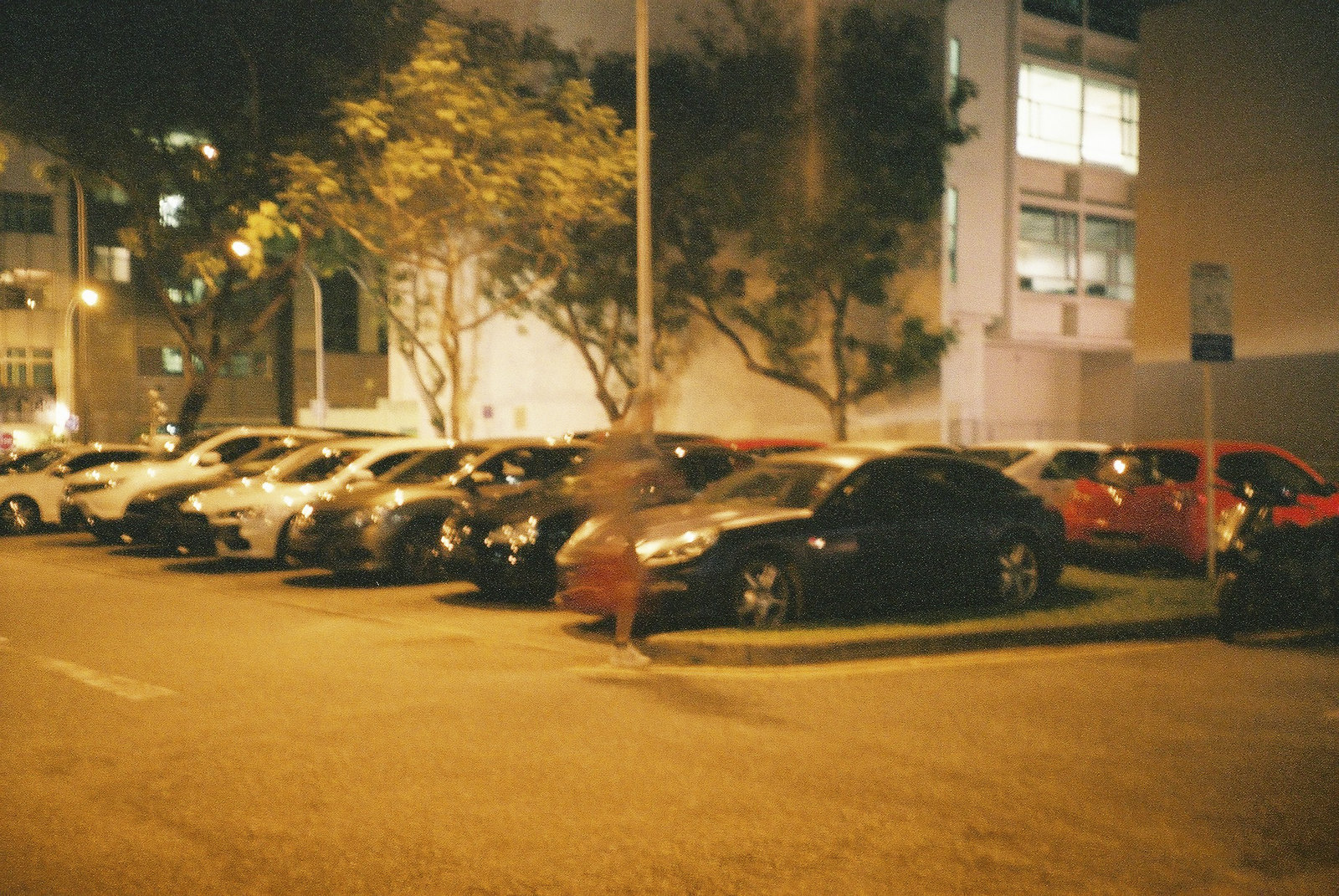The photograph showcases a nighttime scene of a parking lot, presumably belonging to an apartment complex. The primary focus is on an array of cars neatly parked in their designated spots. On the upper right side of the image, extending towards the center, stands a tall, white multi-story building. The building is illuminated with several lights, giving it a slightly luminescent appearance against the night sky. A cluster of trees is partially visible in front of the building, adding a touch of greenery to the scene. In the background, towards the left-hand corner of the image, another apartment building can be seen, contributing to the urban residential atmosphere of the photograph.